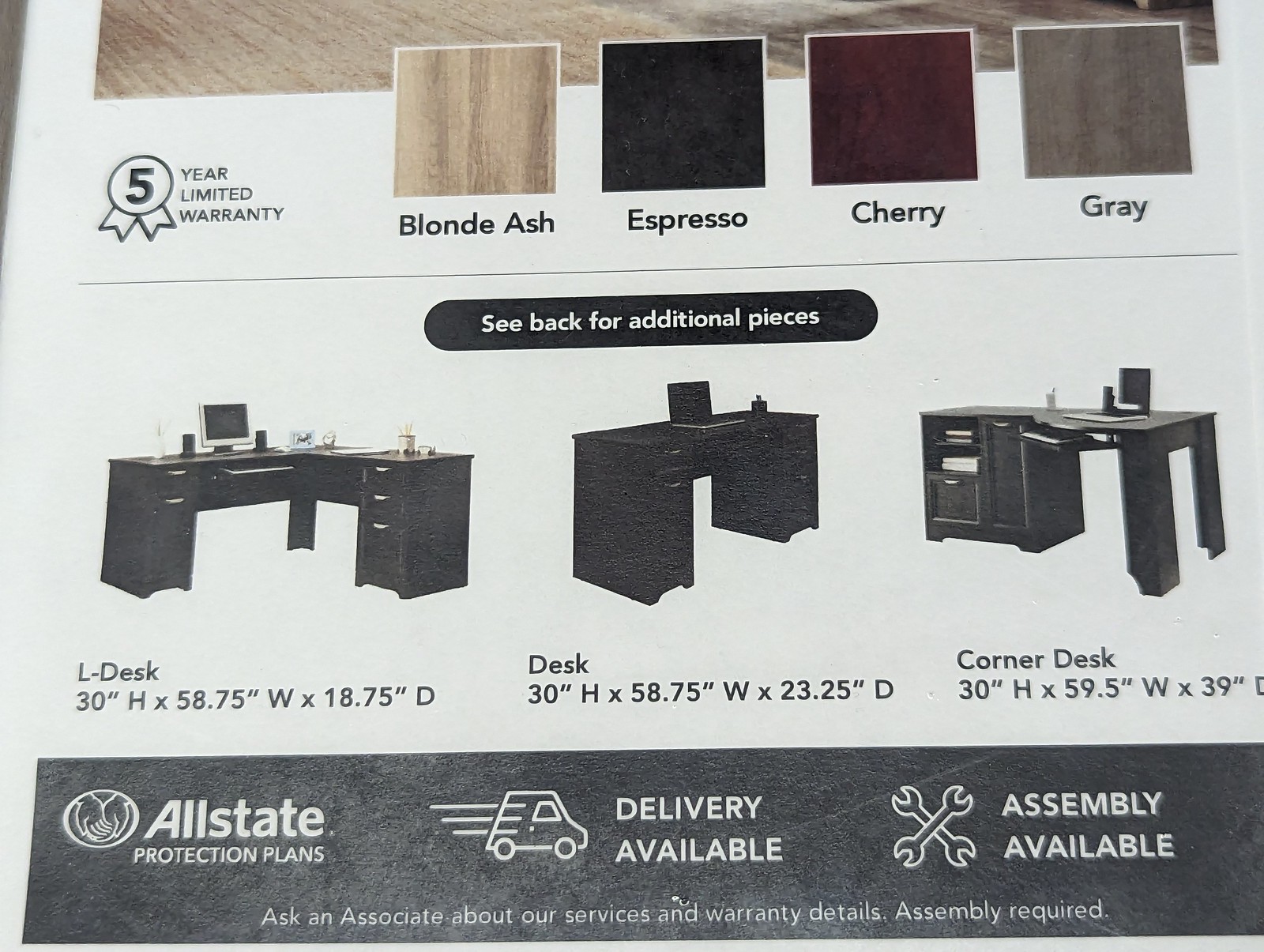This image appears to be an advertisement from a furniture magazine, likely showcasing various desk options and related services. At the top of the image, bold text announces a five-year limited warranty. Below this, four squares display different wood finishes: blonde ash, espresso, cherry, and gray. Each finish is clearly labeled with its corresponding name. 

Beneath the wood samples and to the left, there is a prompt to "see back for additional pieces." This is followed by three black-and-white photographs of different desk types: an L-shaped desk, a standard desk, and a corner desk, each accompanied by detailed dimensions in inches.

Towards the bottom of the advertisement, a black section with white text features additional service options. On the left, the All State protection plans are highlighted, including the recognizable logo of two hands held out. The center highlights delivery services, depicted by a drawing of a speeding vehicle. To the right, assembly services are noted with an illustration of two wrenches crossed in an X. The text emphasizes that assembly is required and encourages readers to ask an associate about available services and warranty details.